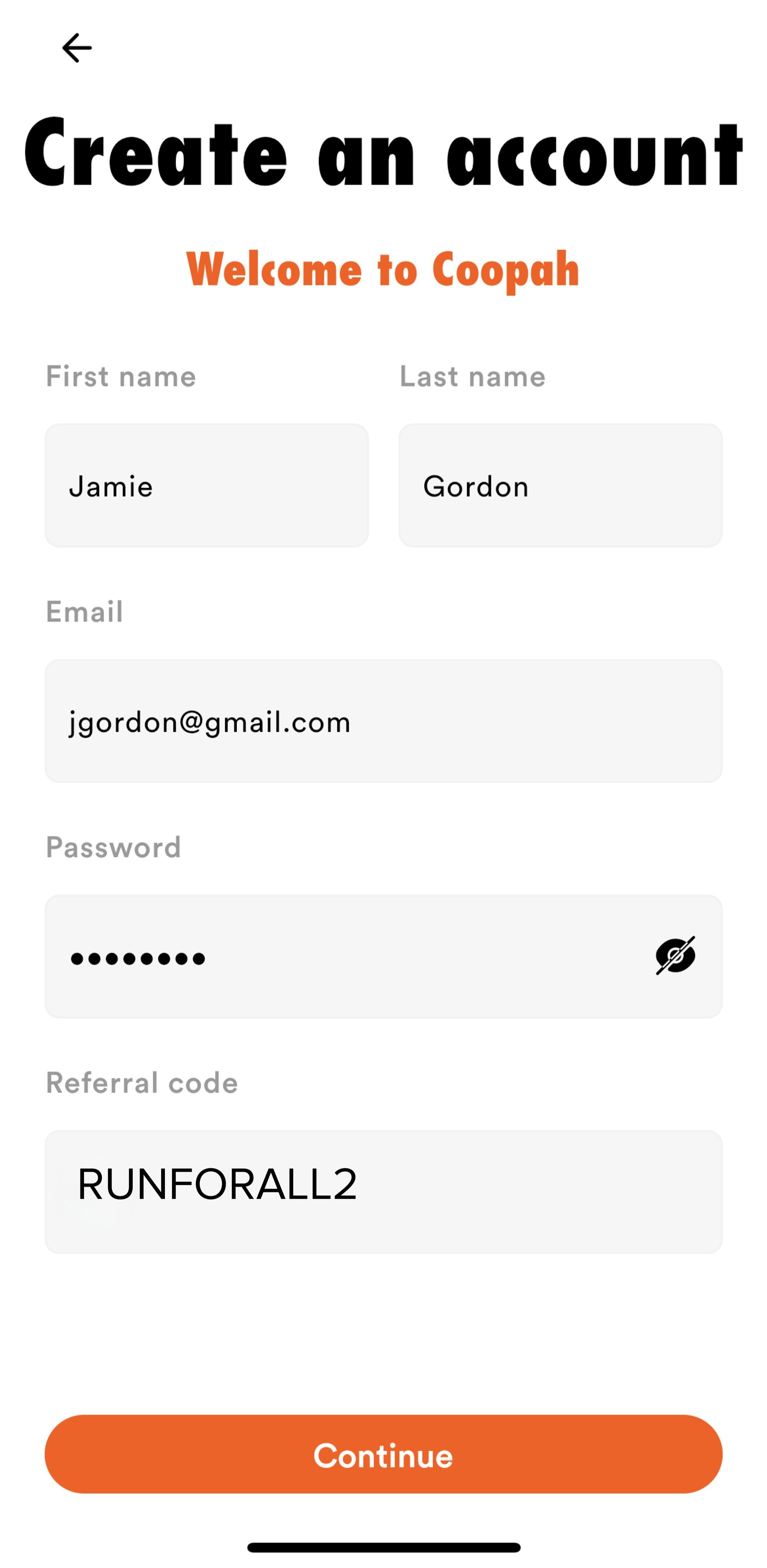The image depicts a smartphone screen showing a "Create an Account" page for an application named "CUPA" (spelled C-O-P-A-H). At the top of the page, "Create an Account" is prominently displayed in bold black text. Below this, the text "Welcome to CUPA" is visible, inviting the user to proceed with the registration.

The form is partly filled out with the following details: In the "First Name" field, the name "Jamie" is entered. In the "Last Name" field, the entry reads "Gordon." The "Email" field contains "jgordon at gmail.com."

The "Password" field is filled with characters represented by seven bullet points, indicating that a password with seven characters has been entered. Adjacent to this field is an icon resembling a black O with a hash line through it, commonly used to toggle password visibility.

Further down, the "Referral Code" field shows the entry "RUN4ALL2" in all capital black letters. At the bottom of the form, an orange button labeled "Continue" is present, ready to be clicked to proceed with the account creation process.